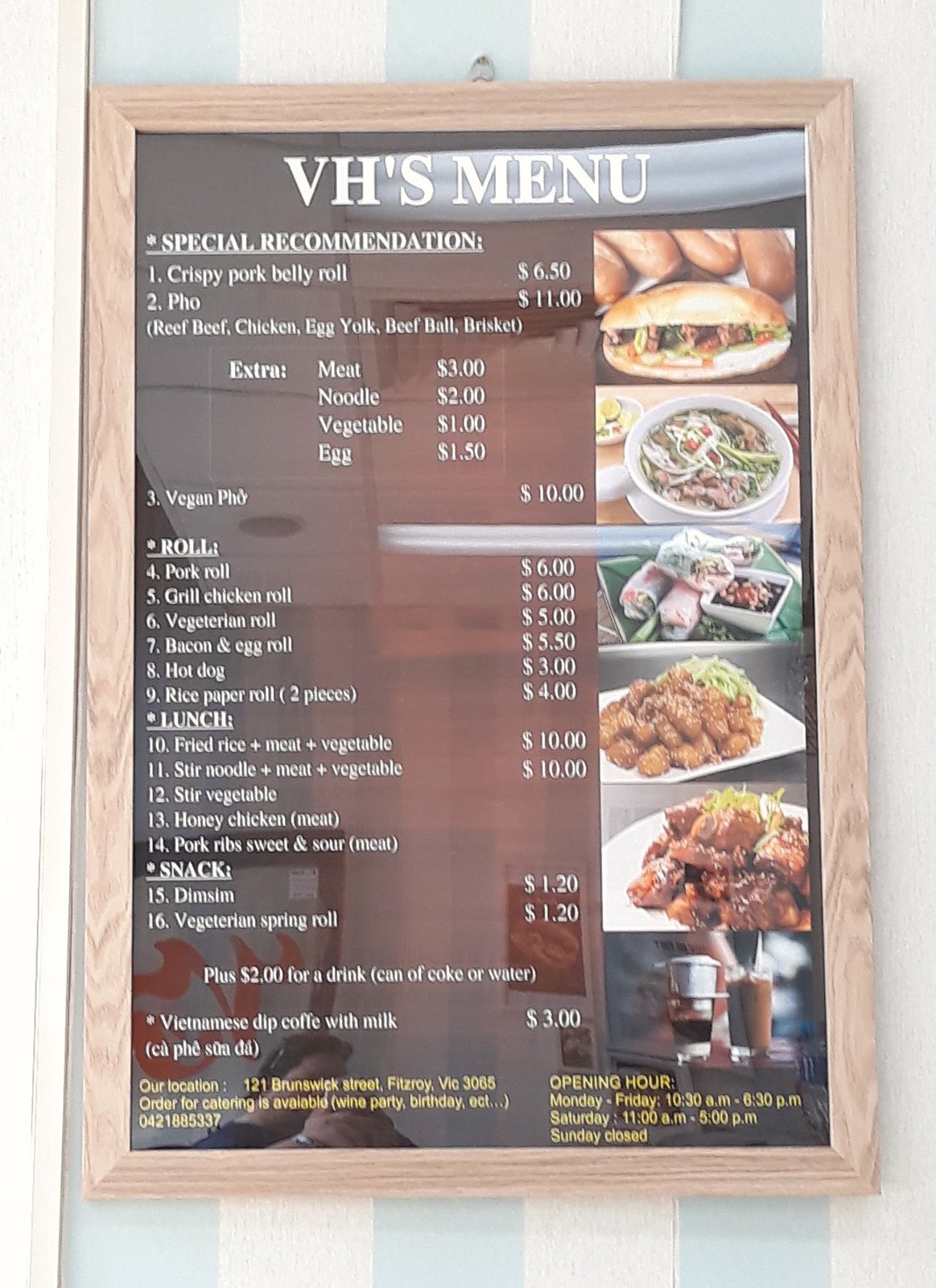The image depicts an elegantly presented restaurant menu displayed within a glossy, magazine-style frame, which is mounted on a wall adorned with light blue, nautical-themed wallpaper. The top of the menu reads "VH's Menu" in dark red lettering.

On the left side of the menu, there is a list of various dishes:

1. **Special Recommendation**:
   - Crispy Pork Belly Roll - $6.50

2. **Pho Options**:
   - Beef Pho - $11
   - Chicken Pho - $11
   - Egg Yolk Pho - $11
   - Beef Ball Pho - $11
   - Brisket Pho - $11
   - Extras: Meat - $3, Noodles - $2, Vegetables - $1, Egg - $1.50

3. **Vegan Options**:
   - Vegan Pho - $10

4. **Rolls**:
   - Pork Roll - $6
   - Grilled Chicken Roll - $6
   - Vegetarian Roll - $5
   - Bacon and Egg Roll - $5.50
   - Hot Dog - $3
   - Rice Paper Roll (2 pieces) - $4

5. **Lunch Specials**:
   - Fried Rice with Meat and Vegetables - $10
   - Stir-Fried Noodles with Meat and Vegetables - $10
   - Stir-Fried Vegetables - $10
   - Honey Chicken - Price not specified
   - Pork Ribs in Sweet and Sour Sauce - Price not specified
   
6. **Snacks**:
   - Dim Sum - $1.20
   - Vegetarian Spring Roll - $1.20
   - Add a drink (Can of Coke or Water) - $2
   
7. **Beverages**:
   - Vietnamese Drip Coffee with Milk - $3

On the right side of the menu, there are photographs showcasing several of the listed dishes, including a sandwich, a bowl of pho, rice paper rolls with various fillings, and close-ups of stir-fried meat dishes and a cup of coffee.

At the bottom of the menu, there are detailed contact and service information, including:

- **Location**: 121 Brunswick Street, Fitzroy, Vic 3065, Canada
- **Catering Services**: Available for wine parties, birthdays, etc.
- **Phone Number**: 042-188-5337

- **Opening Hours**:
   - Monday to Friday: 10.30 am - 6.30 pm
   - Saturday: 11.00 am - 5.00 pm
   - Sunday: Closed

The menu provides a comprehensive overview of the restaurant's offerings along with vivid imagery, making it visually appealing and informative for potential patrons.